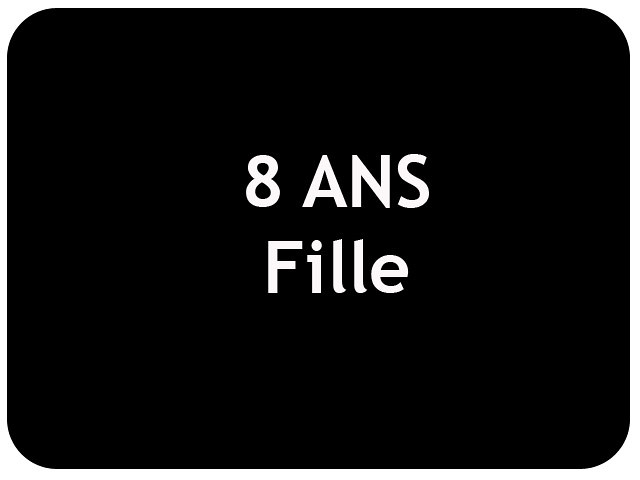The image features a simple, rounded-edge black square, which on some monitors may appear almost dark blue. At the very center of the image, there is a standard white font text displayed in two lines. The first line consists of the number "8" followed by the uppercase letters "A-N-S". Directly below, centered as well, is the word "Fille" with only the "F" capitalized. A close observation reveals slight pixelation around the curves of both the letters and the edges of the black square, suggesting that the image might have been created in Photoshop rather than as a vector graphic. The overall aesthetic is straightforward with no additional elements or background distractions.